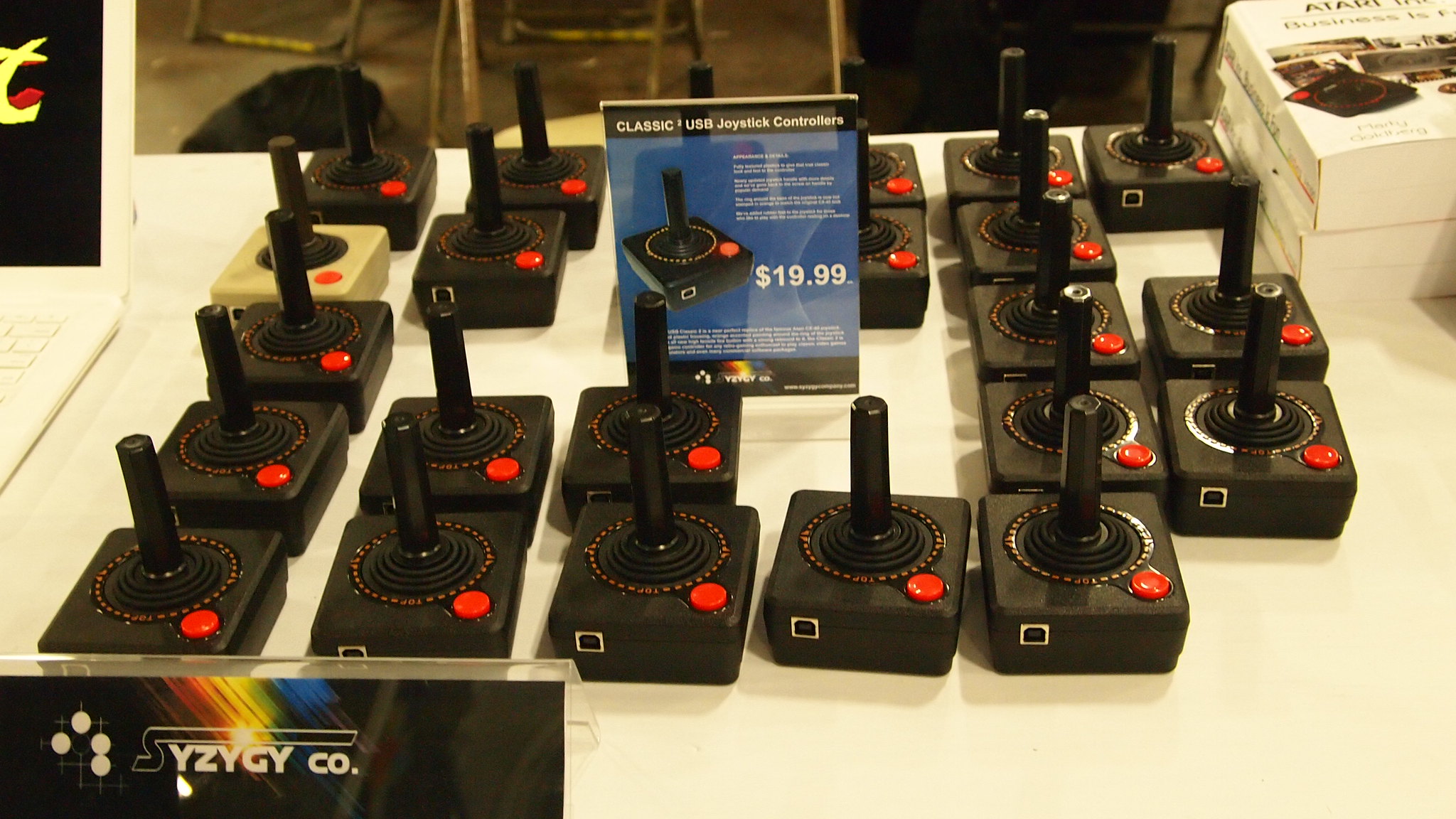This photograph captures a vintage collection of approximately 20 Atari video game controllers meticulously arranged in a rectangular formation on a white table. These classic controllers are predominantly black with a distinctive joystick and a red button, except for one cream-colored variant near a laptop with a black screen in the top left corner. Central to the image is a blue sign featuring an image of the controller, the text "Classic USB Joystick Controllers," additional unreadable white text, and a price tag of $19.99. At the bottom right corner of the table, a black sign with a rainbow motif reads "Syzygy Co." Additionally, in the upper right corner, there are two thick white books, one mentioning "Atari" and "Business." The neat, grid-like arrangement of the controllers and the inclusion of the sign and laptop create a visually organized and informative display of these nostalgic gaming devices.